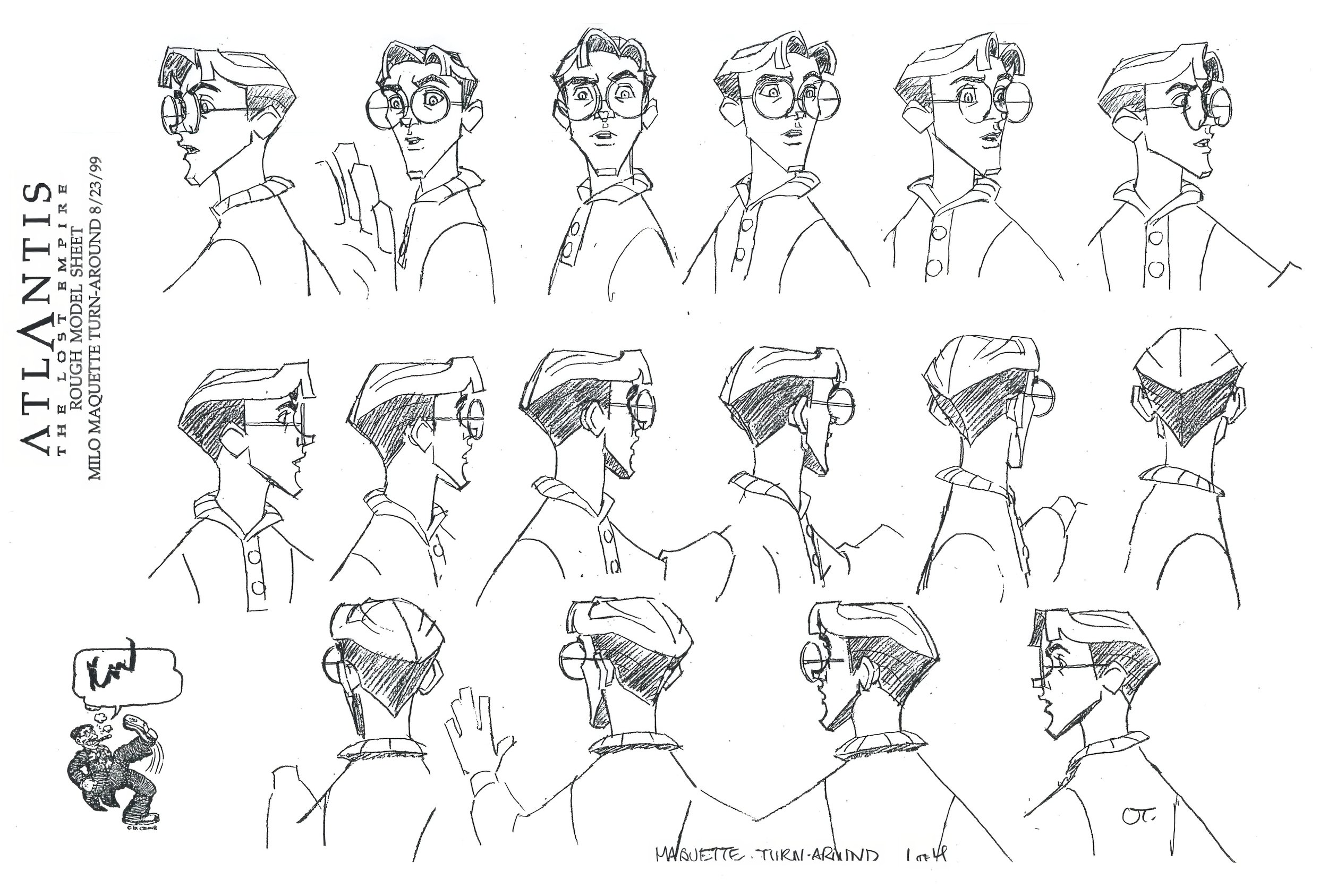This detailed black-and-white pencil sketch serves as a rough model sheet for the character Milo from the animated movie "Atlantis: The Lost Empire." It features approximately 15 to 20 drawings of Milo displayed across three rows, capturing every possible angle of the character. In the top row, Milo is depicted mostly facing forward with a look of awe or curiosity, enhanced by his big round glasses. As the sketches progress down to the second and third rows, Milo is shown turning to his left, ultimately revealing the back of his head in the bottom row. He has swept-back hair, and wears a partially buttoned collared shirt. Additionally, there's a small drawing of a character resembling Groucho Marx with a cigar and a foot kicked in the air at the bottom. On the left side of the sheet, written vertically, are the texts "Atlantis: The Lost Empire," "Rough Model Sheet," "Milo Maquette," "Turnaround," and "V-23, 1999." The entire sheet appears to be a preliminary concept to practice or finalize the design of Milo for the movie.